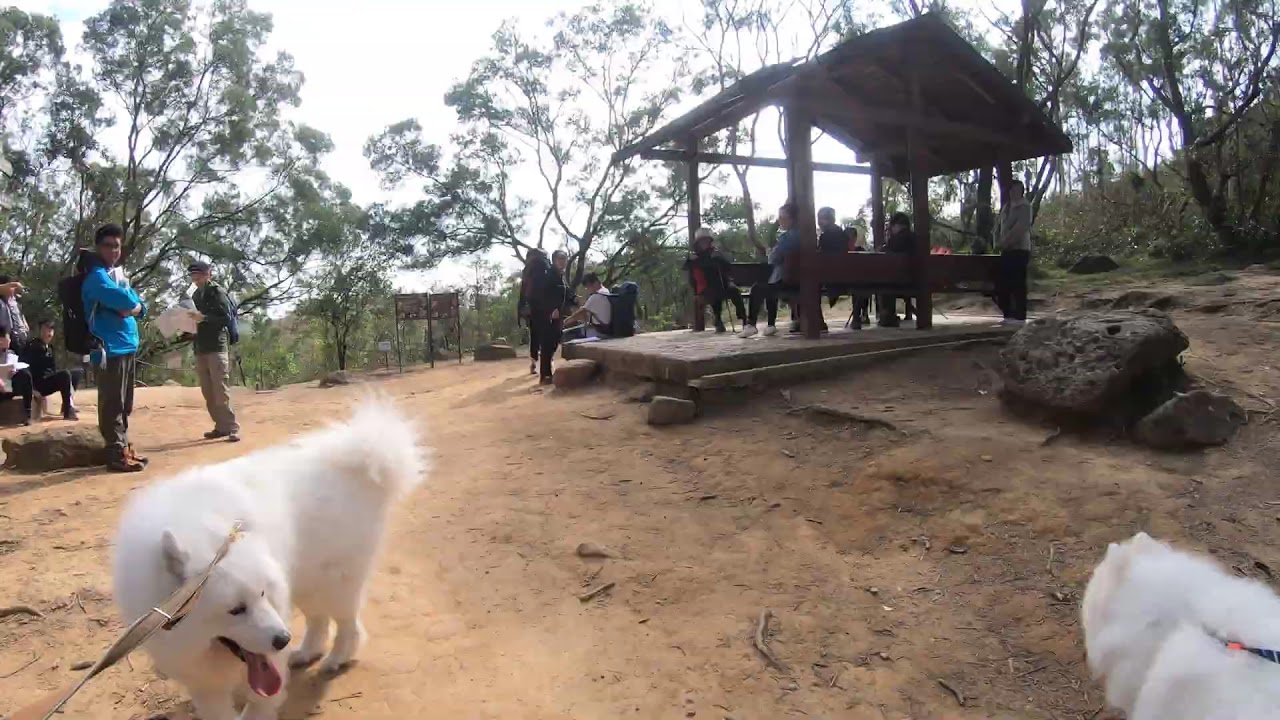The image captures a scenic overlook situated within a dirt-covered natural environment, likely part of a state or national park. In the foreground, two large white dogs on leashes are positioned at opposite corners—one on a black leash to the bottom right, and the other on a tan leash to the bottom left. On the right side, a prominent large, porous boulder is accompanied by a smaller boulder. The center top reveals a wooden structure with posts and a covered roof, providing shelter to various people sitting on the benches beneath. The individuals scattered throughout the image are equipped with hiking backpacks, tennis shoes, and travel attire, indicating a day trip. The sky is a light gray, devoid of clouds, adding a subdued backdrop to this busy, well-trodden overlook area.